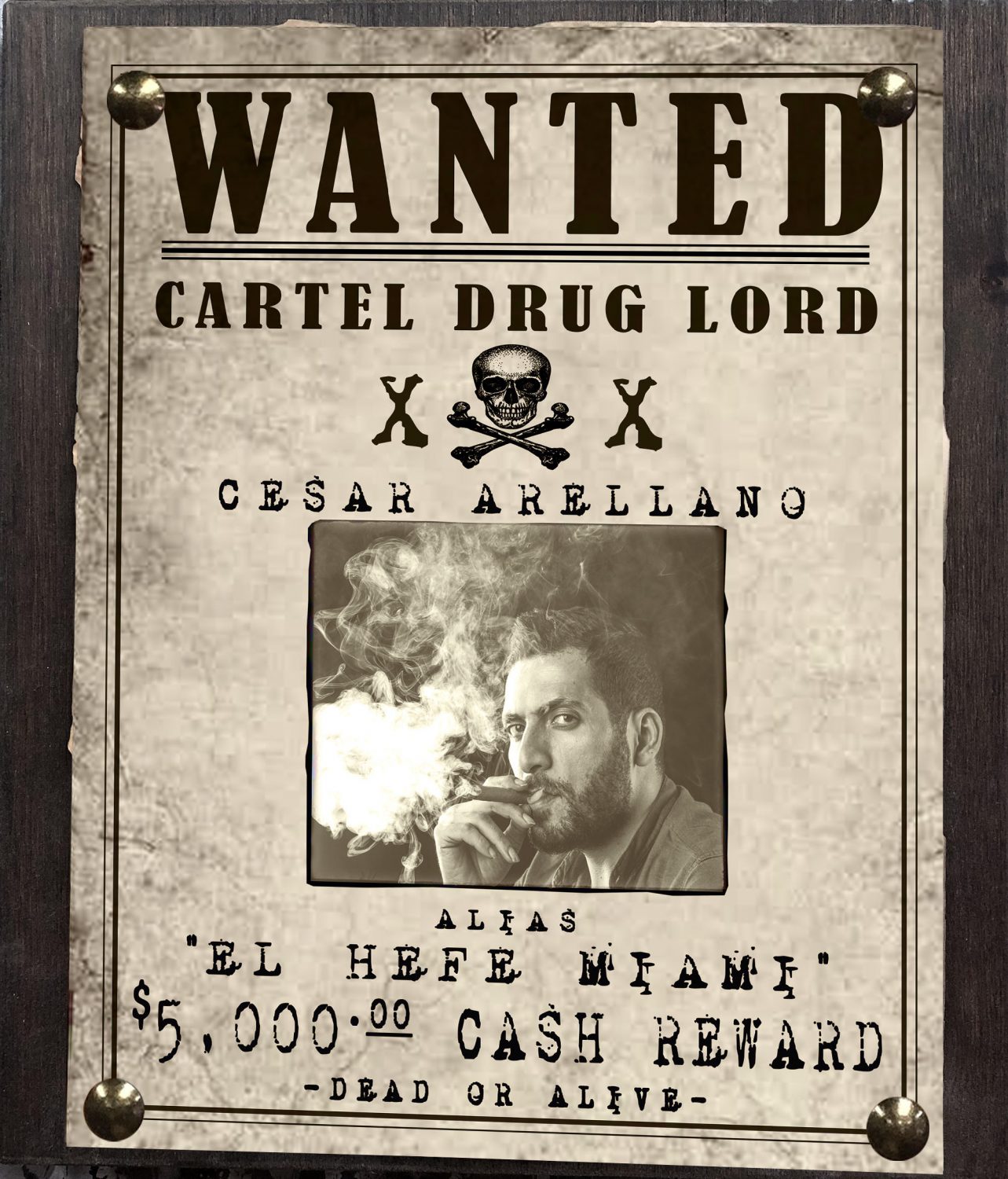The image is a vintage-style wanted poster prominently reading "WANTED" in bold, all capital letters at the top, followed by "CARTEL DRUG LORD" beneath it. Between these lines, a drawn skull and crossbones are situated. Below this, the name "Cesar Arellano" is displayed, with a black-and-white portrait of him smoking a cigar directly underneath, a light puff of smoke visible against the dark gray background. Cesar Arellano has short dark hair and a black goatee. Under the photo, in typewriter font, it reads "Alias: El Jefe Miami," followed by "$5,000 Cash Reward," and "Dead or Alive," all in black text. The poster appears to be attached to a board using four round, silver rivets, one in each corner.